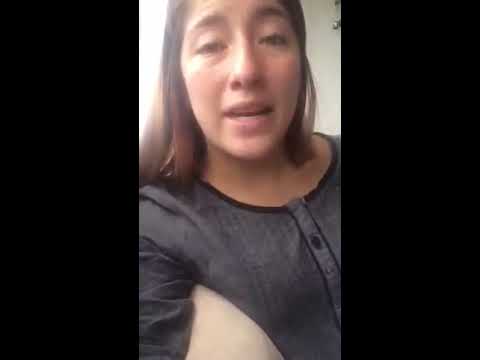This close-up digital photograph captures a woman in her 30s with shoulder-length brown hair and a slight tan, mid-sentence with a surprised expression on her face. She is wearing a dark gray, long-sleeved button-up blouse with a black collar and black buttons. Her right arm is in front of her, possibly holding a pillow under her right arm, where a white area is visible. The background is stark white, and the image has blacked-out sections on the left and right, emphasizing the rectangular visible area in the middle. Light from the room creates a slight glare on the right side of her face, adding to the detailed atmosphere of the scene.